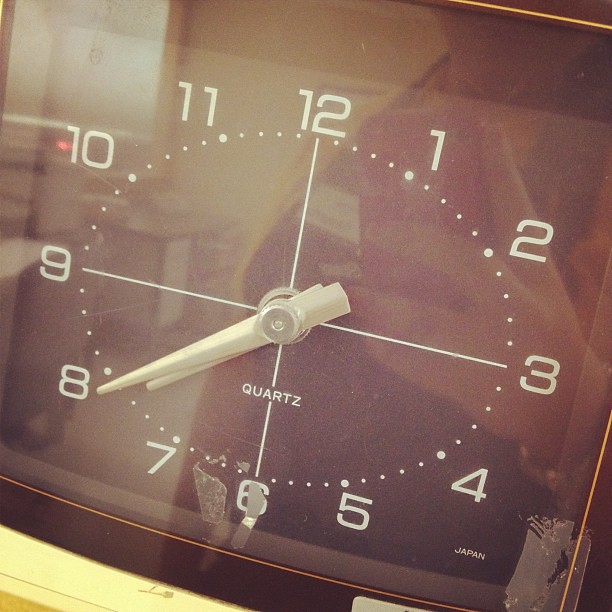This photograph captures a detailed, close-up view of a square clock face resting on a light-colored surface, visible in the bottom left corner. The clock's outer rim is a sleek black, accentuated with a thin gold line encircling the face. The face itself is black, with white numerals elegantly marking the hours. Small dots represent the minute markings, with slightly larger dots underscoring each five-minute interval. The clock hands are a crisp white, and just below their meeting point at the center, the word "quartz" is prominently displayed. In small, white lettering, the word "Japan" is inscribed in the bottom right corner of the clock face. Notably, there are remnants of adhesive marks in the bottom right and center bottom regions, suggesting the previous presence of tape or a sticky substance.